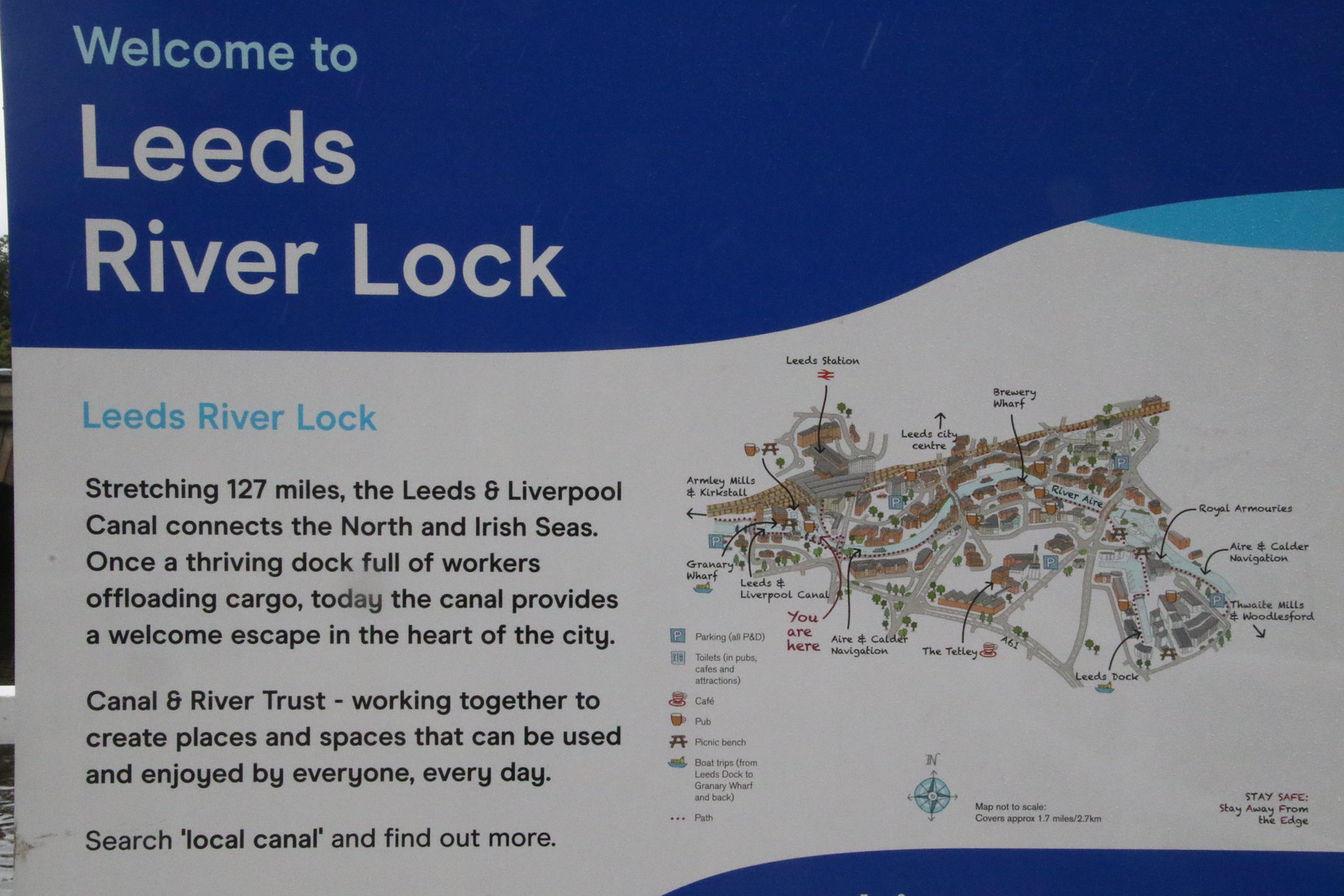This image captures an outdoor informational sign for Leeds River Lock. On the left side, the text reads: "Welcome to Leeds River Lock. Leeds River Lock, stretching 127 miles, the Leeds and Liverpool Canal connects the North and Irish Seas. Once a thriving dock full of workers offloading cargo, today the canal provides a welcome escape in the heart of the city. Canal and River Trust, working together to create places and spaces that can be used and enjoyed by everyone, every day. Search local canal, find out more." The text is presented against a white background, with the heading set against a blue background. To the right of the text is a detailed map marked with various locations and symbols, including pubs and other notable features. The map also includes a compass indicating directions. The photo appears to have been taken during the daytime, and some elements of the surrounding outdoor environment are visible on the left side of the image.